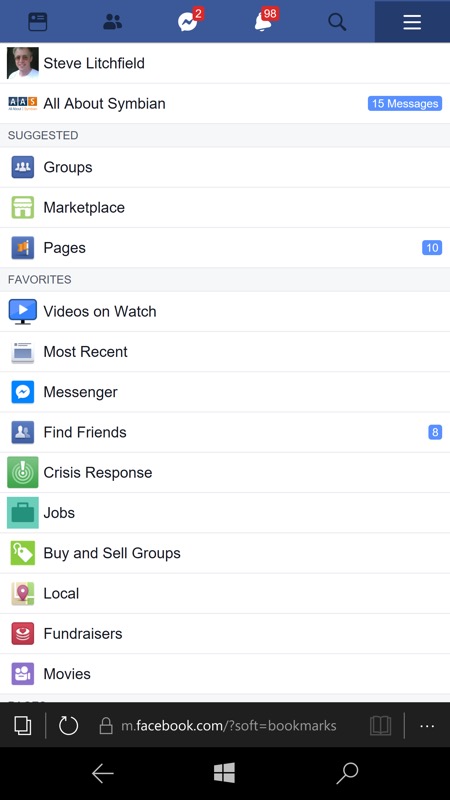At the top of the image, there is a long blue bar, featuring a small white circle with a lightning bolt icon in it. Directly above this icon in a red circle is the number "2". To the right of the lightning bolt is a bell icon, with the number "98" in a red circle beside it. This interface appears to be from Facebook.

Below the blue bar, there is a profile image of a man wearing sunglasses, who has gray hair and is dressed in a white t-shirt. The name "Steve Litchfield" is displayed next to the profile image. Directly below the name is the text "All about Symbian". To the right of this text, inside a blue square, is the number "15" indicating messages.

Further down, the word "Suggested" is followed by several subcategories which include "Groups," "Marketplace," and "Pages." Beside "Pages", in a blue square, is the number "10". The next subcategory is "Favorites."

Below this, a list of options includes "Videos on Watch," "Most Recent," "Messenger," "Find Friends," "Crisis Response," "Jobs," "Buy and Sell Groups," "Local," "Fundraisers," and "Movies." Right of the "Find Friends" option is a small blue square.

At the very bottom, inside a search bar, "facebook.com" is shown, likely indicating a URL, along with "soft bookmarks." To the right is another search bar, and in the bottom left corner, there is a left arrow icon.